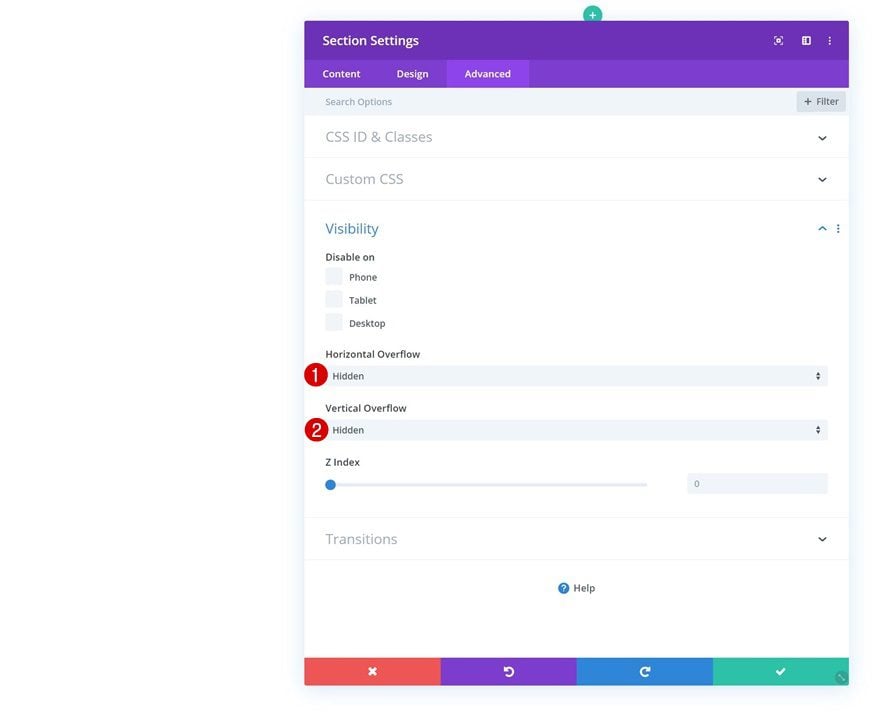Sure, here is a cleaned-up and detailed caption for the image:

---

The image showcases a user interface design with various settings options. At the top, there is a purple header set against a white background, displaying the text "Section Settings" in white. Below the header, there is a green circle with a white plus sign. The interface is divided into three main tabs: "Content," "Design," and "Advanced," with "Advanced" currently highlighted against a gray background, distinguishing it from the other two tabs which have a purple background.

Under the "Advanced" tab, there are multiple customizable options:
1. A blue rectangle labeled "Search Options."
2. A gray rectangle featuring a "Filter" option alongside a plus sign.
3. An area detailing "CSS ID and Classes" and a section for "Custom CSS."
4. Visibility settings with three checkboxes labeled "Phone," "Tablet," and "Desktop"; all of them are marked as disabled.
5. Horizontal overflow settings displayed in a box labeled "Hidden," accompanied by a red circle with the number 1 in white.
6. Vertical overflow settings also in a box labeled "Hidden," with a red circle showing the number 2 in white.
7. A section for setting the Z-index, featuring a bar with a blue circle positioned at the far left side and a gray rectangle displaying the number 0.
8. Transition settings with an arrow pointing downwards.
9. A help icon, represented as a blue circle with a white question mark inside it.
  
At the bottom of the section, there are four rectangles, each featuring different colors, perhaps indicating additional settings or status indicators.

---